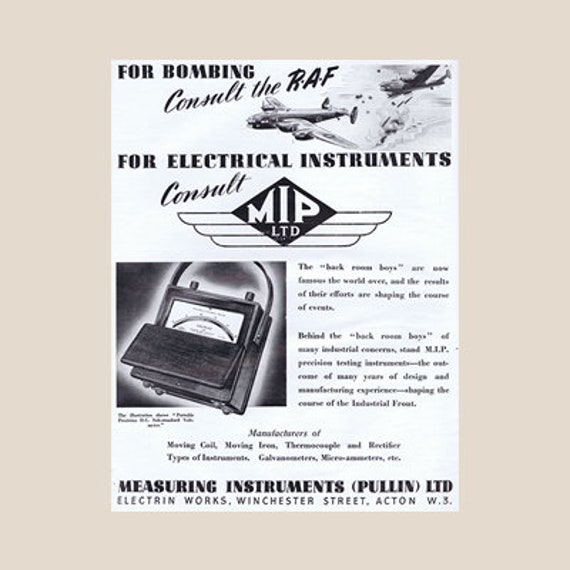This black, white, and gray poster, likely from the 1940s, serves as an advertisement for electrical instruments made by MIP Limited. The top of the poster features dramatic imagery of RAF warplanes engaged in combat, accompanied by the text, "For bombing, consult the RAF." Below, it states, "For electrical instruments, consult MIP Limited," drawing a parallel between the precision needed in wartime efforts and the reliability of the company's products. The right side of the poster contains paragraphs detailing the company's offerings and the high quality of their instruments, while at the bottom, it lists "Measuring Instruments, Pullin Limited, Electric and Works, Winchester Street." A detailed illustration of an electrical instrument, possibly a meter or similar device sold by the company, is prominently featured, further emphasizing the company's technical expertise. This poster blends wartime patriotism with commercial promotion, suggesting a symbiotic relationship between military efforts and industrial innovation.